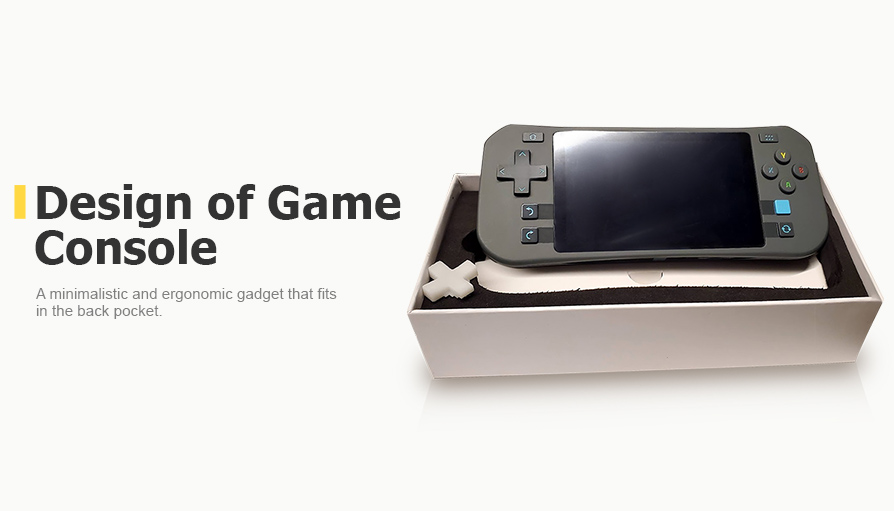This image showcases a modern handheld gaming console that combines sleek design with ergonomic functionality. The centerpiece of the image features a black handheld gaming device with a central oversized flat LCD screen. On its left side, there is a cross-shaped directional pad with arrow buttons at each corner. On the right side, there are four distinct round buttons marked with letters—Y in yellow, X in blue, A in green, and B in red. Below the main controls, additional blue buttons for navigation and a black square button are visible. The gaming device sits atop a glossy white box lined with foam, providing a pristine and safe enclosure. Text on the white background includes bold black letters stating, "Design of a Game Console," followed by a gray subtext reading, "A minimalist and ergonomic gadget that fits in the back pocket." The image's clean and minimalist style emphasizes both the innovative design and the portability of the handheld gaming console.